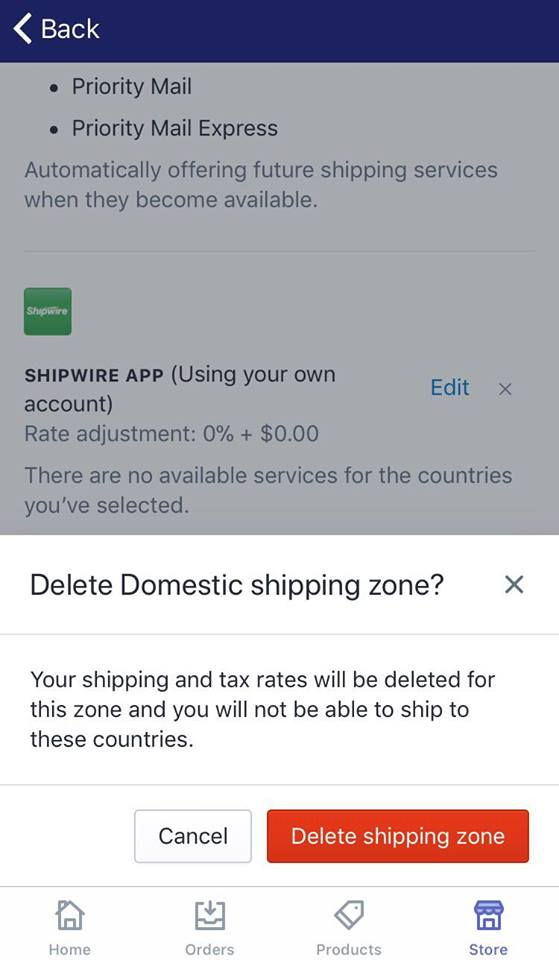This screenshot, taken from a mobile device, features a vertically oriented image. At the very top, there is a thin navy blue strip with the word "Back" in white text pointing to the left. Beneath this strip, there is a gray box containing text. The top of the gray box displays two bullet points: "Priority Mail" and "Priority Mail Express." Below these bullet points, a note states, "Automatically offer future shipping services when they become available."

Further down, a small green box with "Shipwire" in white text is visible. Directly beneath this box, the text "SHIPWIRE APP" is written in black, capital letters, followed by a parenthetical note: "(Using your own account rate adjustment 0% + $0.00)."

A gray notice at the bottom of the box reads, "There are no available services for the countries you've selected." To the right of this notice is a blue "Edit" option.

The remainder of the image has a white background with the text "Delete Domestic Shipping Zone" accompanied by an "X" on the right side. Below this, it states, "Your shipping and tax rates will be deleted for this zone, and you will not be able to ship to these countries." Towards the bottom, there are two buttons: a white "Cancel" button on the left and an orange "Delete Shipping Zone" button on the right, both with white text.

Finally, at the very bottom of the screen, there are four navigation icons labeled "Home," "Orders," "Products," and "Store." The "Store" icon is highlighted in blue, indicating it is currently selected.